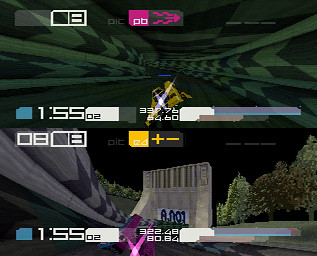This image features a screen capture from a vintage video game, depicting a dark outdoor scene. Dominating the lower center is a gray concrete wall, which curves off towards the left side of the image. Above, a green, metallic roof stretches across the upper portion of the scene, creating a sense of depth and perspective. In the middle section, black shadows envelop a brown and green spaceship-like structure. Overlaying the scene, a bar runs horizontally across the center, displaying the time 1:55:02. The topmost section of this bar reads "08," which is repeated directly below the time. Additional timestamps, "1:55:02," "3:22:48," and "80.84," are present at the bottom of the image, likely representing various game scores or statistics.